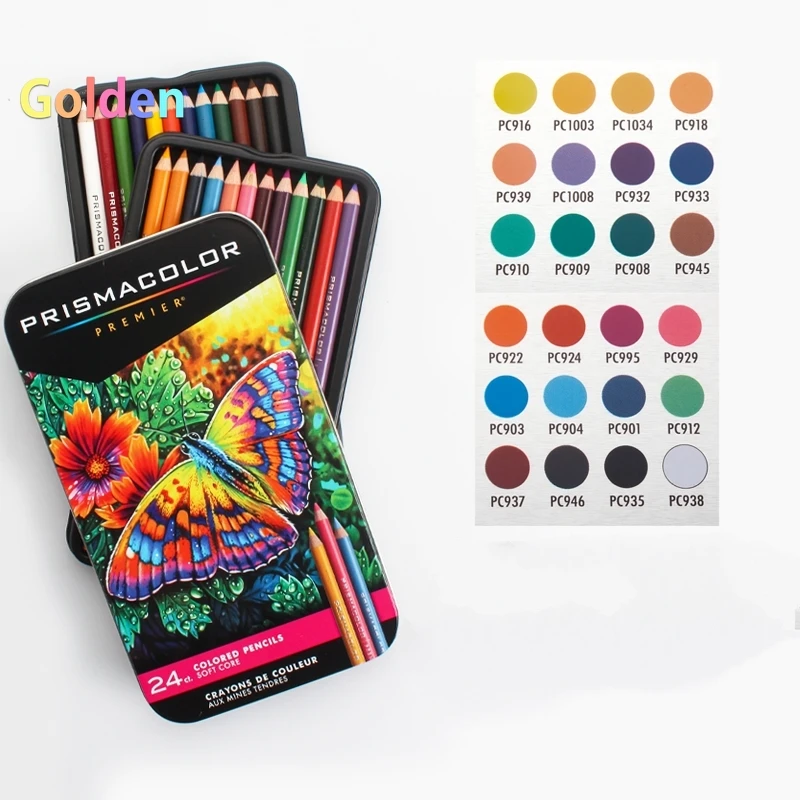The image showcases an open box of Prismacolor Premier colored pencils, prominently featuring the word "GOLDEN" on the left-hand side in various colors. This boxed set contains 24 vibrant colored pencils. The box itself includes a detailed, hand-drawn illustration of a butterfly with wings adorned in hues of yellow, purple, blue, and pink, perched on dew-kissed flowers with green leaves and a red-purple center. The butterfly and flowers embody the rich color possibilities within the Prismacolor set. To the right of the image, a comprehensive color chart displays all the available shades in the set, ranging from white, black, red, and blue, to maroon, teal, purple, yellow, and various shades of gold and brown. The image captures the vibrant and diverse color palette these premium colored pencils offer, illustrating both their artistic potential and quality.